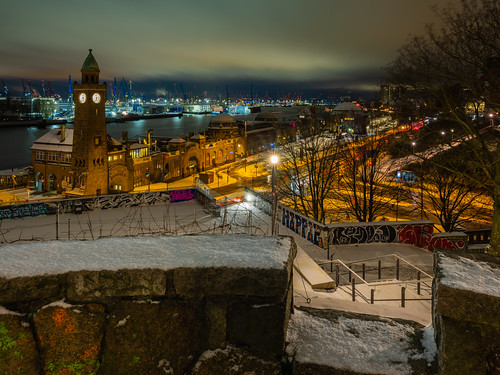This detailed nighttime aerial photograph captures a vibrant cityscape from a high vantage point. In the foreground, a stone balcony, dusted with snow, offers an elevated perspective overlooking a diverse urban landscape. Below, a snow-covered stone fence adorned with various graffiti descends towards a main street flanked by smaller buildings. Prominently, a historic church with an illuminated clock tower stands tall to the left, its architectural details sharply contrasted against the wintry scene. 

To the right, trees frame the view, partially obscuring roadways where cars traverse illuminated by streetlights and billboards. Beyond the clock tower, a serene river reflects the city's lights, separating the historic section from a modern cityscape visible in the distance, shimmering under a slate blue night sky. The city's intricate network of streets and cross streets is interlaced with patches of snow-covered parkland, and occasional railings, adding depth and texture to the scene.